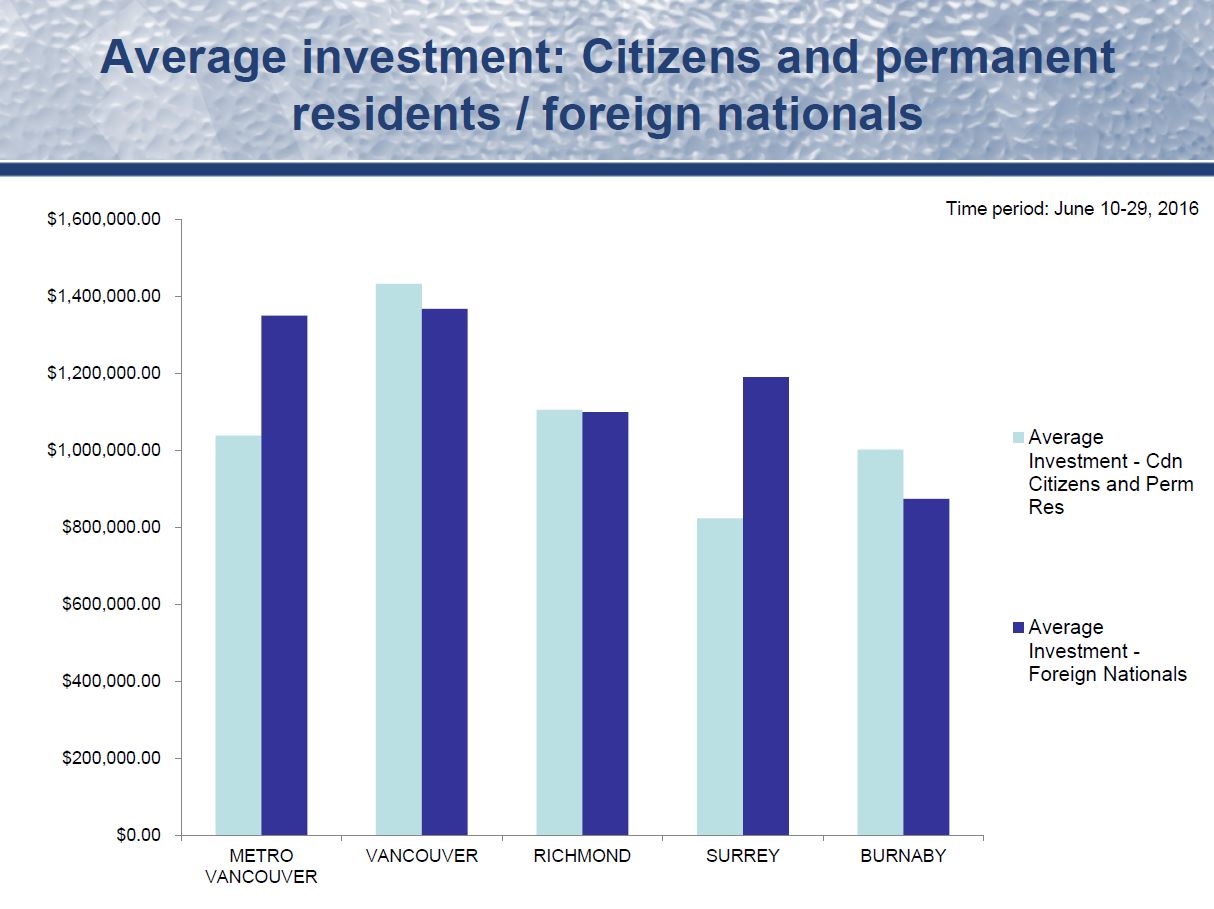The image displays a bar chart titled "Average Investment, Citizens and Permanent Residents / Foreign Nationals" in dark blue text, positioned on a hammered gray background at the top of the chart. The vertical axis on the far left enumerates values from 0 to 1.6 million in intervals of $200,000. The horizontal axis categorizes different regions in Canada: Metro Vancouver, Vancouver, Richmond, Surrey, and Burnaby. Key legends denote that light blue bars represent the "Average Investment for CDN Citizens and Permanent Residents," while dark blue bars signify the "Average Investment for Foreign Nationals." The chart indicates that in Metro Vancouver, foreign nationals invest more than citizens and permanent residents, while in Vancouver, the reverse is true. In Richmond, both groups have similar investment levels. In Surrey and Burnaby, citizens and permanent residents have higher investments than foreign nationals. The time period for this data spans from June 10th to June 29th, 2016.